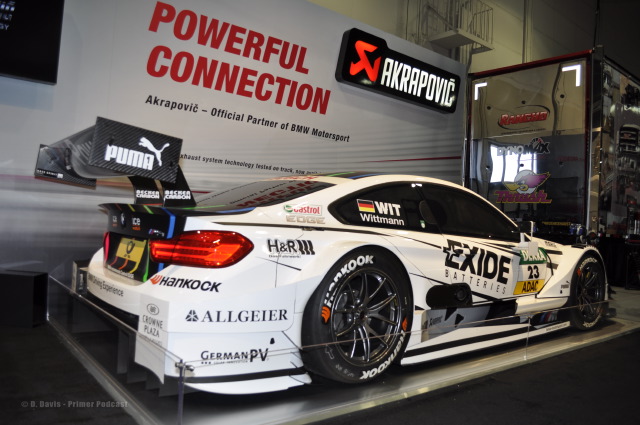A white race car is exhibited on a plastic stand, encased by short, clear plexiglass barriers that extend up about a quarter of the car's height. The car features black tinted windows and is adorned with numerous advertisements. Prominently, "Exide Batteries" is displayed on the door, "H&R" is marked on the rear fender at the top, and "LG'er" and "German PV" are marked on the rear fender at the bottom. Below the headlight, the word "Hankook" appears, which is also branded on the tires. The car sports a black spoiler on the back, emblazoned with "Puma" on the top. Behind the car, a large white sign reads "Powerful Connection," with a banner in red stating "Akrapovic, Official Partner of BMW Motorsport." Additionally, there is a lit-up sign featuring a red crescent-shaped item and "AKRAPOVIC" inscribed beside it.